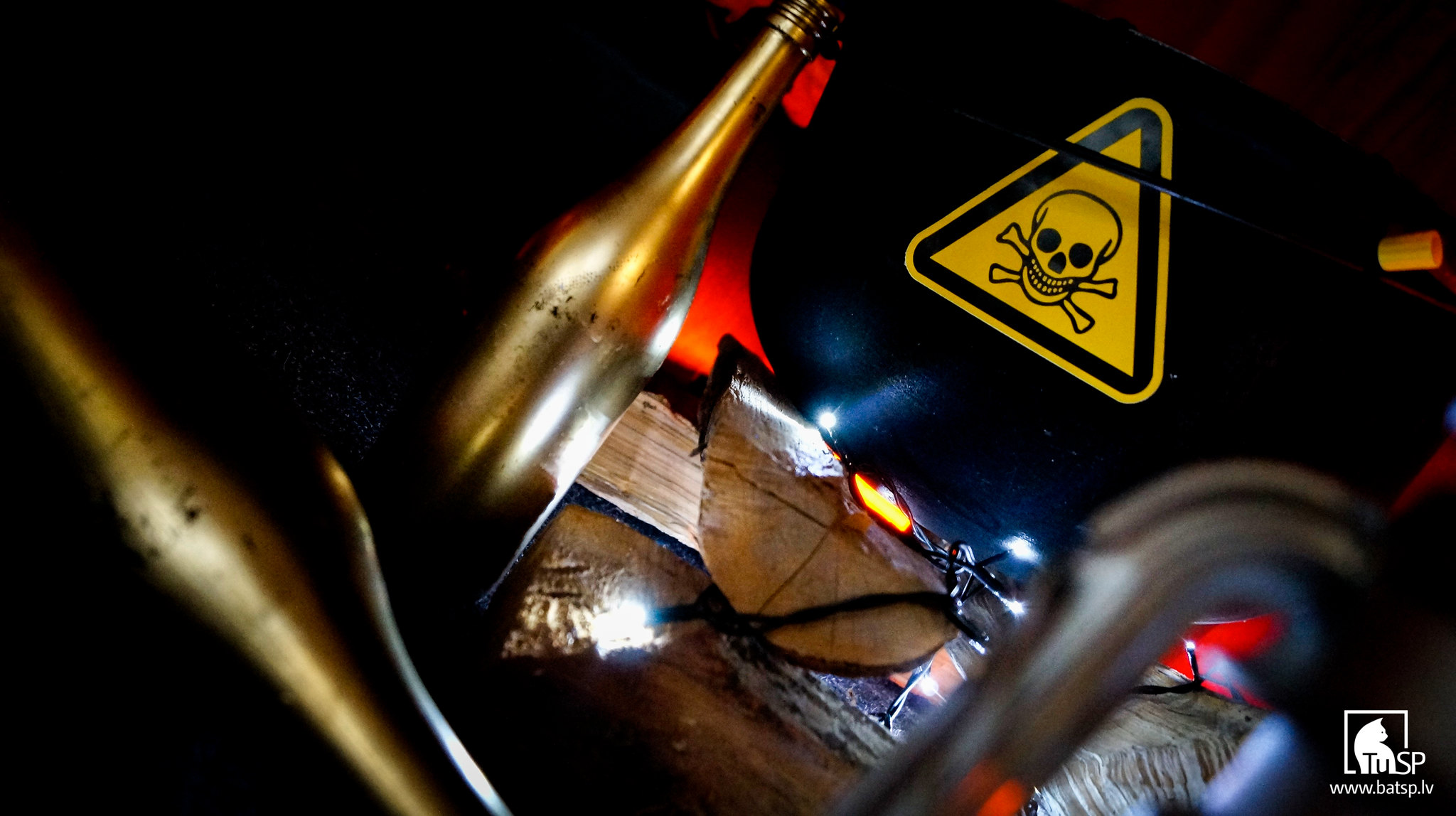The image features two metal, silver, screw-top bottles, one standing upright and the other lying horizontally beneath it. Positioned slightly above to the right in the background is a yellow warning sign outlined in black. The sign displays a black skull and crossbones, with a small black triangle located above the skull, creating a secondary yellow triangle within the larger one. The scene is blurred, making it difficult to discern precise details. The entire background of the image is black. In the bottom right-hand corner, there's a logo depicting a bear inside a white box, with the text "T-U-S-P" and a website address, "www.batsp.lv."